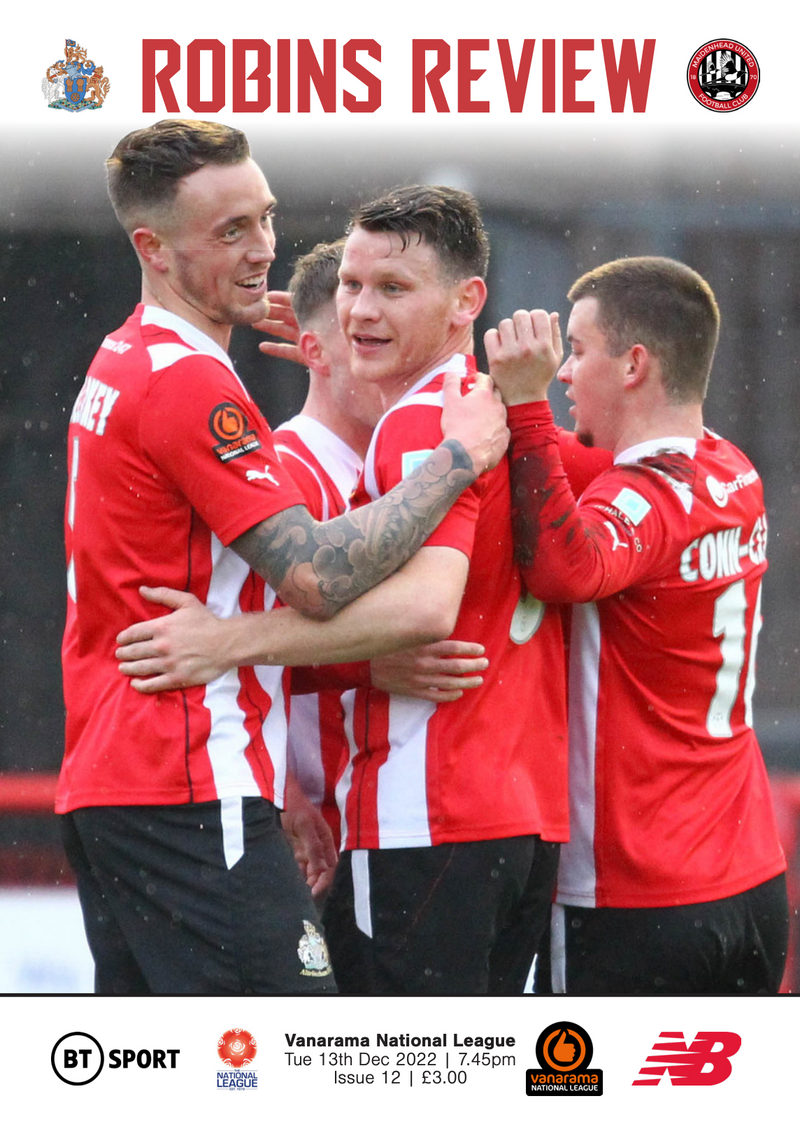This tall rectangular poster for a sports event prominently features a photograph that occupies most of the space, depicting four male athletes with white skin and short brown hair, some of which is longer on top but buzzed on the sides. They are huddled closely together, wearing red shirts with white stripes and black shorts adorned with white lines. The leftmost athlete stands out as the tallest and has tattoo-covered arms. Above them, at the top of the poster, in bold red letters on a white background, it reads "Robbins Review". This title is flanked by two logos: a coat of arms featuring a lion on the left and a red and black circular design on the right. The image is subtly accented with what appears to be white snow droplets. Below the players, another white portion features an array of advertisements, including references to BT Sport, the National League, Vanarama National League, and a New Balance (NB) logo, along with details indicating it is issue 12 of the Robbins Review magazine, priced at three pounds.